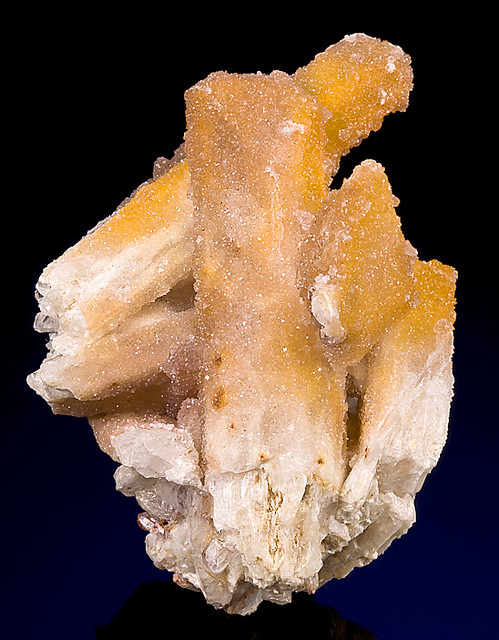The close-up photograph showcases a striking rock formation that resembles a fossilized heart or a geode, set against a predominantly black background with a subtle blue tint in the bottom right corner. The geode-like rock is highly detailed, exhibiting crystalline structures that are mostly orange and brown, transitioning to a beige color towards the bottom. The formation features several jagged, vertical structures emerging from a white, ball-like base, with one central pillar ascending vertically and another extending diagonally near the top. The entire piece, which sparkles with a quartz-like texture, appears to be mounted on a black stand, highlighting its intricate and multi-faceted crystal composition.